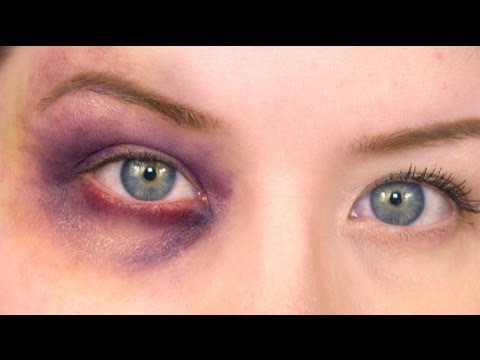This highly detailed photograph captures a close-up of a woman's face, focusing exclusively on her eyes, eyebrows, and the bridge of her nose. The woman has beautifully manicured, thin eyebrows and pale, European-like skin. Her eyes are striking, described as a blue-gray or hazel that seem to convey a direct, clear expression despite the severe bruising. The left eye is the focal point, exhibiting a painful-looking black eye with extensive bruising in multiple hues—dark purple, red, yellow, and brown—that encircle the eye and extend above her eyebrow. The bruising is especially dark and pronounced under her eye and at the outer edges. She has mascara on her right eye, but her left eye lacks any, further accentuating the injury. The image reveals a small amount of acne near the top right of her forehead, adding to the raw and unshielded portrayal of her face.